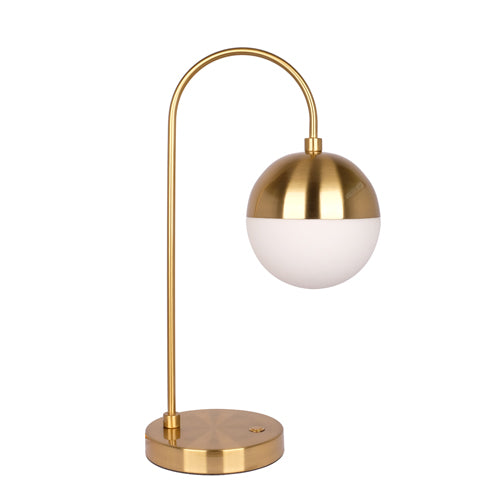This vertical image captures a modern, highly polished lamp with no visible boundaries. The lamp's base is a small, circular disc in a reflective brass color, featuring a very thin, small button to turn it on and off. A thin metal rod, inserted through a thick washer or bolt, extends vertically from the base, bends 180 degrees in a U-turn or candy cane shape, and faces downward. Hanging from the end of the rod is the lamp's spherical head, where the top half matches the brass material of the pole and base, and the bottom half is a transparent white acrylic or plastic. Light reflections are visible on both the base and the top part of the spherical head, with two small squares on the base and two longer squares on the brass portion of the head. The lamp is set against a white background, photographed with professional lighting to emphasize its sleek and modern design.